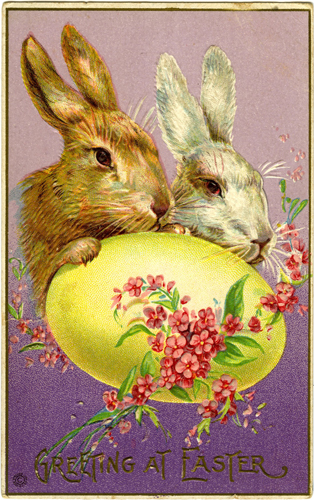This detailed Easter photograph showcases a hand-drawn artwork inside a light gold picture frame with a mauve background. The drawing features two caricatured bunnies, one white and one brown, with wicked-looking eyes. Both bunnies are peering over a large yellow egg adorned with a wreath of flowers, which combines pink shrubs and red flowers intertwined with a green vine. The scene is set against a gradient background that transitions from dark purple at the bottom to light purple at the top. The bottom of the image has golden engraved writing that reads "greeting at Easter," making it clear that this is an Easter card or themed artwork.